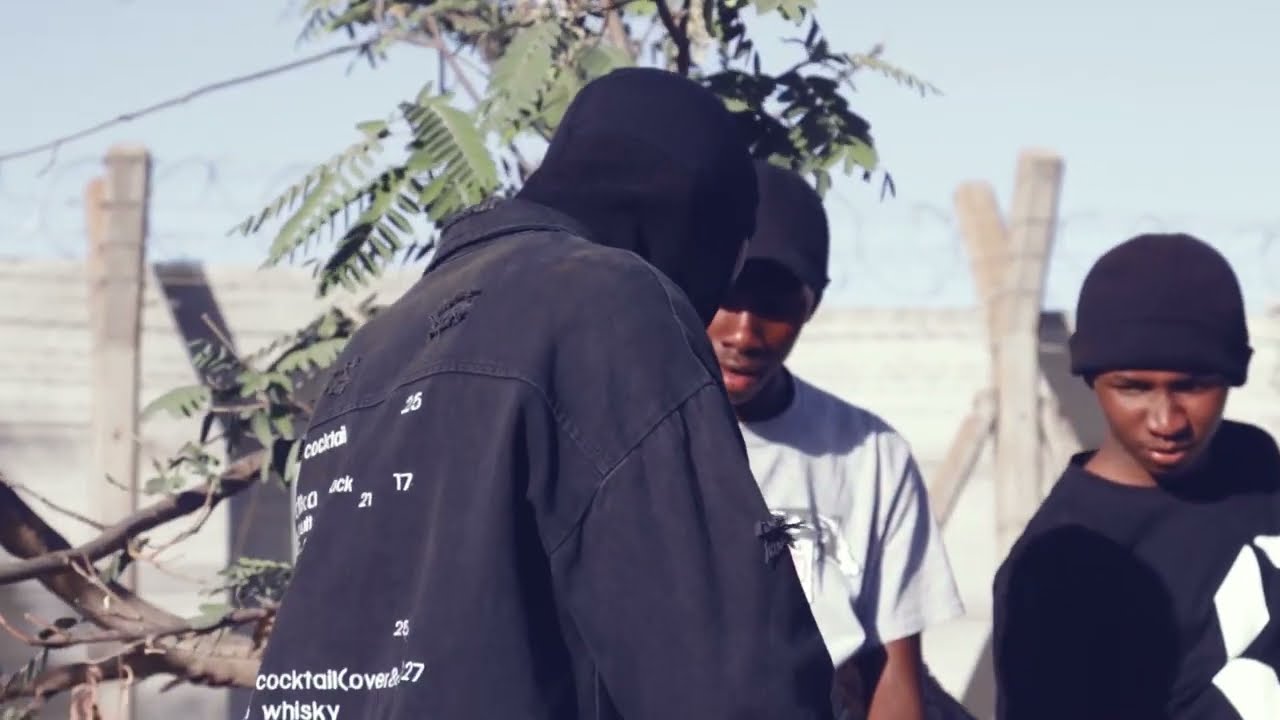The photograph captures an outdoor scene on a clear day, featuring three young black males. In the foreground, there's a male turned away from the camera, wearing a black hood and a tattered black denim jacket with white text that reads "Cocktail Cover Whiskey." His face is obscured by a black mask. To the right, partially blocked by the hooded figure, stands a black male in a white t-shirt and black baseball cap. Next to him, another black male in a black t-shirt with a white logo and a black stocking cap is present. Both of these individuals are looking down at an object that the hooded figure is holding, although the object itself is not visible in the photo. The backdrop includes a tall barbed wire fence with wooden poles and layers of razor wire, suggesting a confined or secure area. Trees and green leaves add a touch of nature to the otherwise stark environment.